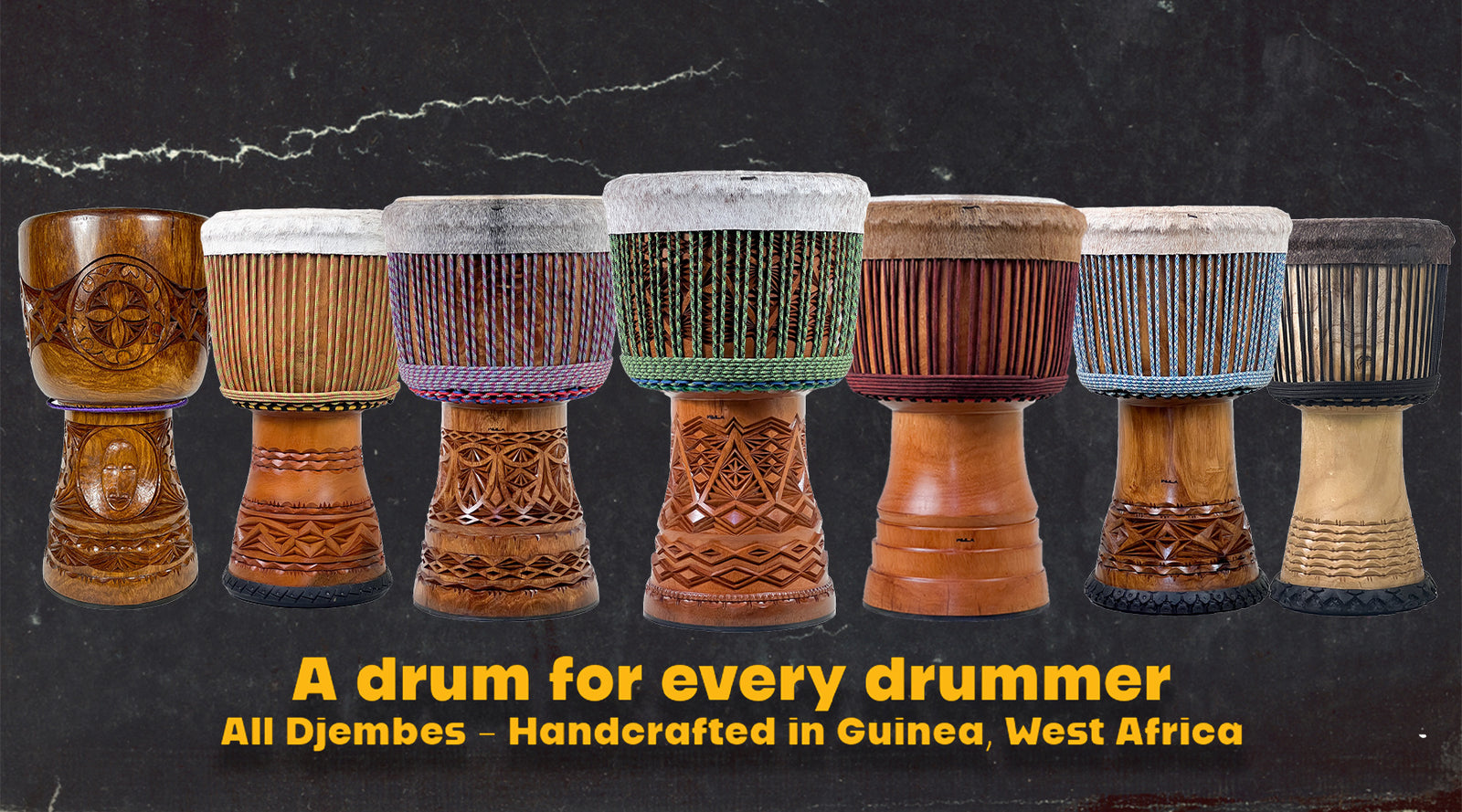This image features a detailed advertisement for handcrafted djembes, African drums that originate from Guinea, West Africa. Enjoying a black marble-like background, the foreground showcases seven exquisitely hand-carved wooden djembes, each flaunting unique embossed iconography and intricate imagery. The drums are fabulously lacquered and polished, with wood hues ranging from deep brown to orange and a lighter cream color. 

Each djembe sports a traditional skin or leather top, varying in shades from white and gray to rich brown and deep black. Some also feature colorful beadings and embroideries: blue and pink embroidery with a purple finish, green and white beading, or blue and brown ropes. Notable is the drum on the left, adorned with a lotus-like flower and a face elegantly painted into its varnish, distinguishing it from the others. 

A prominent yellow text at the bottom of the image reads, "A drum for every drummer. All djembes handcrafted in Guinea, West Africa," emphasizing the authenticity and artistic craftsmanship of these musical instruments.